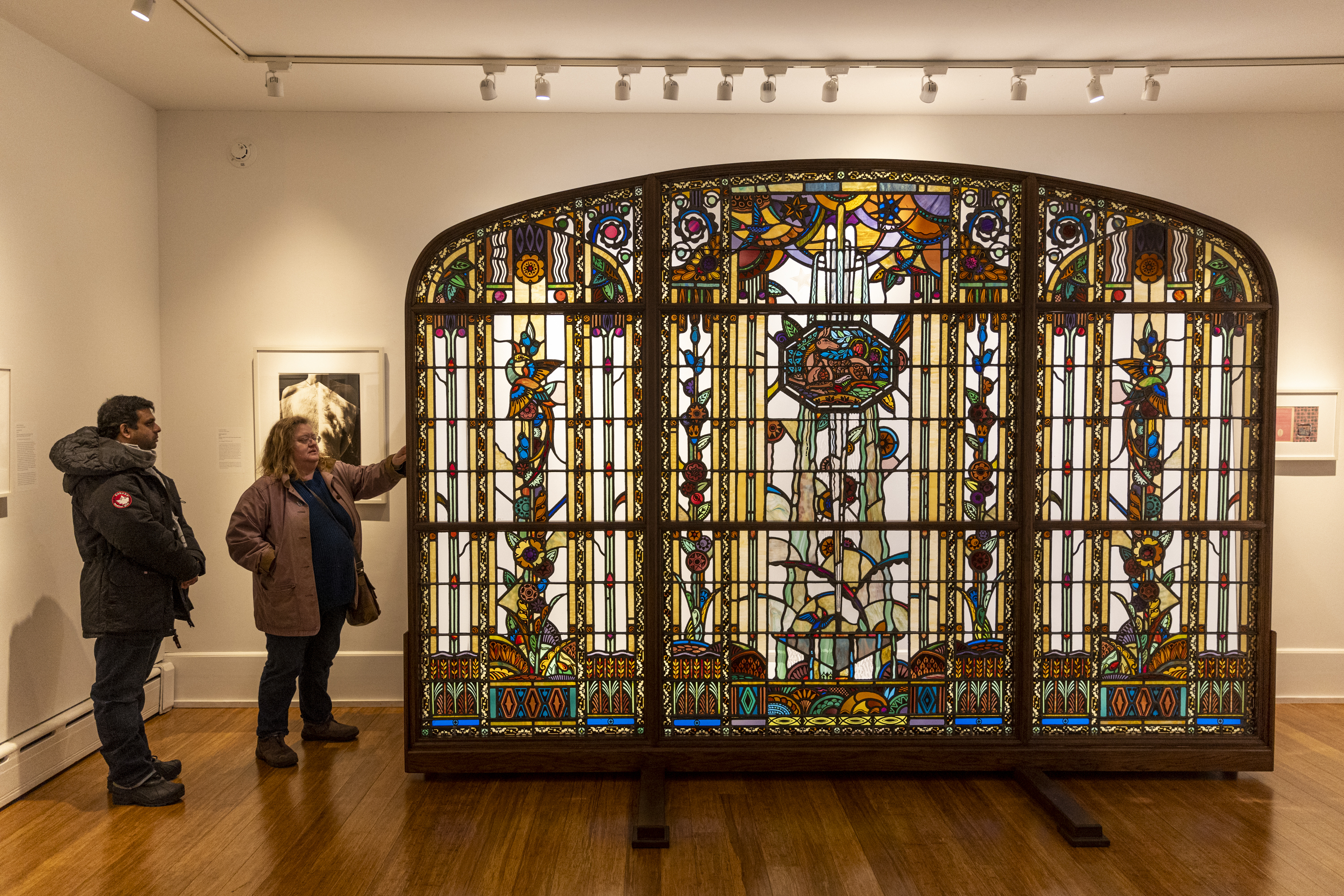The image captures a stunning stained glass window prominently displayed inside an art gallery or exhibition space. The window, set up under a strip of 13 spotlights mounted on the ceiling, is the focal point of the room. This magnificent piece is encased in dark wood framing, dividing it into three vertical panes, further segmented into nine smaller sections with a beautifully curved top edge. The intricate design features a floral motif in a rich palette of colors, including yellow, blue, orange, purple, red, turquoise, and subtle touches of brown and white.

In the scene, the stained glass window stands on a wooden stand against a backdrop of a clean, white wall adorned with two framed paintings, one on each side of the window. The gallery has a shiny wooden floor that adds a touch of elegance to the setting.

To the left of the window, two individuals, a man and a woman, are admiring the artwork. The woman, dressed in a beige jacket, black top, dark trousers, brown shoes, and carrying a handbag over her left shoulder, appears to be reaching out and touching the stained glass. Her mid-length blondish hair contrasts with the man's darker attire. The man, with brown skin color, wears a parka jacket, casual clothing, and stands beside her with his hands in his pockets, observing the intricate details of the window. Both individuals are dressed warmly, indicating a winter season.